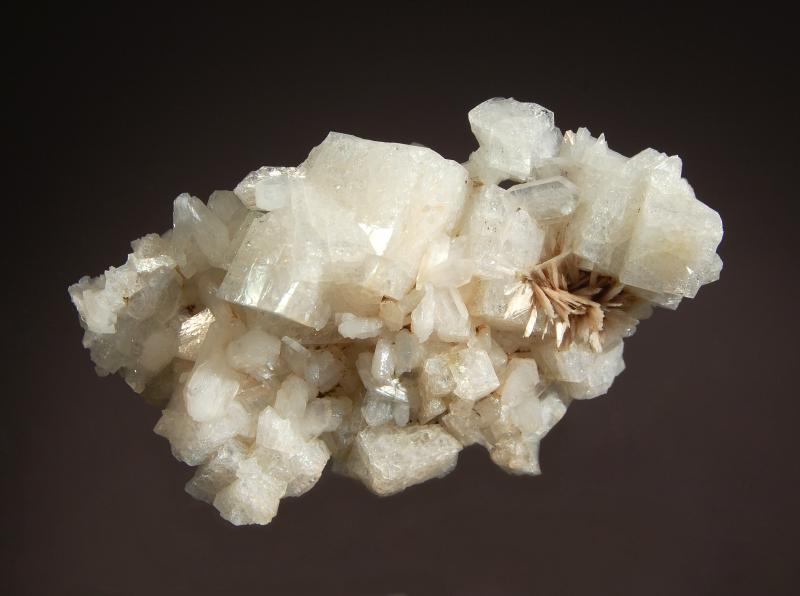This photograph showcases a striking clump of crystallized rock, predominantly composed of off-white to white crystals with subtle yellow tinges. The main structure is a conglomerate of smaller, squarish crystal formations that create an intricate, larger piece. The texture varies, with areas that are both shiny and grainy, adding to the visual complexity. On the right side, there are distinct, spiky protrusions with a tan hue, potentially a different type of mineral or crystal. The image is taken in close-up, enhancing the details of the crystals. The background is a black gradient, transitioning from a lighter shade in the center to darker edges, with the light source seemingly originating from the bottom right. This detailed setting highlights the unique textures and formations of the crystals.